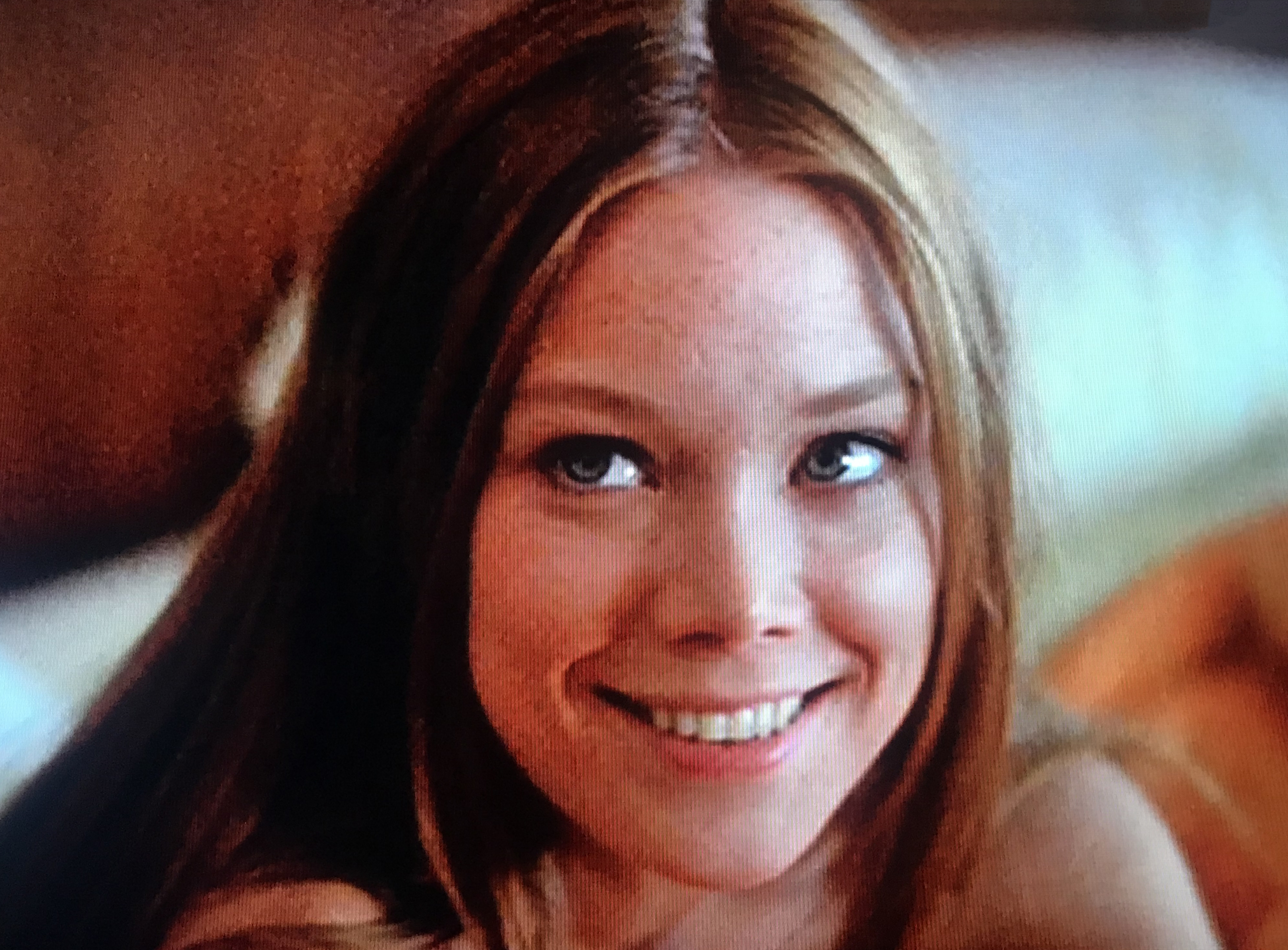The image displays a young woman with long, middle-parted brown hair, and her facial expression combines a grin with slightly rolled eyes as she looks up to the left. Light freckles dot her fair skin, and her eyes appear a mix of light colors, possibly brownish-green. She is shown from the shoulders up, and it is ambiguous whether she is wearing a top, giving a subtle implication of nudity. She is sitting on an orange couch, with a backdrop that includes an orangish-brown wall to the left and a white object, possibly a table, behind her. The overall scene has a vintage vibe reminiscent of the 1970s, enhanced by scan lines that give it a retro, possibly film still-like appearance. The background is blurry, focusing attention on her expressive face and smile.